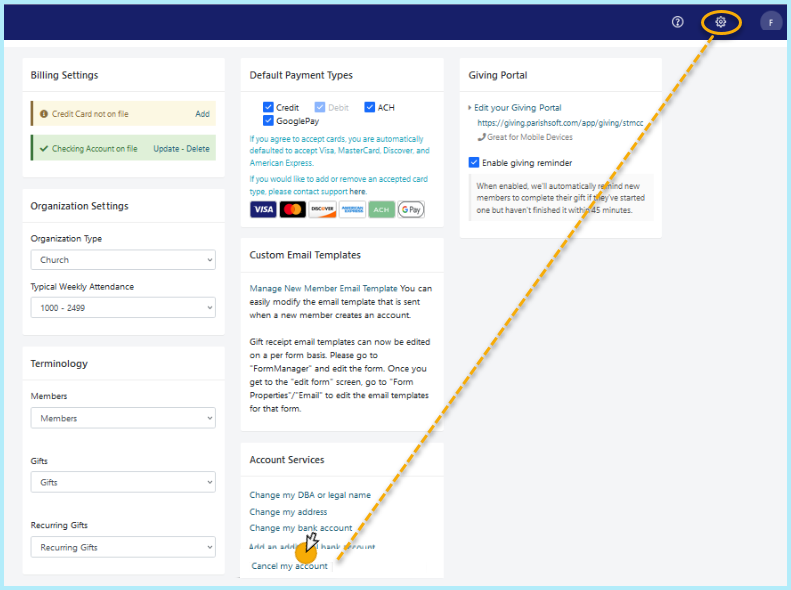**Caption: Detailed Layout of Website Billing and Organizational Settings**

The website features a three-column layout dedicated to various settings and configurations. 

**Column One: Billing Settings**
- **Header:** The header is highlighted with a blue bar and features a settings icon. 
- **Settings Details:** 
  - **Credit Card Status:** Indicates that no credit card is currently on file, with options to add, update, or delete a credit card.
  - **Organization Settings:**
    - **Organization Type:** Church
    - **Typical Weekly Attendance:** $1,000 to $2,499 
    - **Terminology Used:** Members
    - **Gifts and Recurring Gifts:** Defined simply as "gifts" and "recurring gifts."

**Column Two: Default Payment Types**
- The section outlines the available default payment options:
  - **Accepted Payment Types:** Credit, ACH, Google Pay
  - **Credit Card Networks:** Visa, MasterCard, Discover, and American Express are automatically enabled.
  - **Modification:** For adding or removing any card types, users are advised to contact support.
- **Payment Icons:** Visual icons for Visa, MasterCard, Discover, Amex, ACH, and Google Pay.

**Column Three: Custom Email Templates**
- **Management:** 
  - Users can manage and customize email templates.
  - **New Member Email Template:** Editable template for welcome emails when a new member creates an account.
  - **Gift/Receipt Email Templates:** These can be customized on a per-form basis. Users are directed to the form manager for template editing.

This detailed arrangement ensures users have clear, organized access to their billing and organizational preferences, making it easier to manage settings and communication templates.